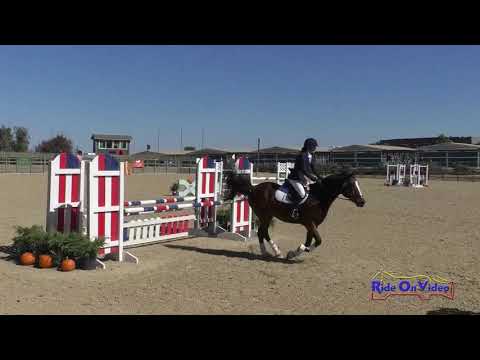In this detailed outdoor image, a professional rider, likely a jockey, is captured mid-action while riding a black-brown horse with a white blaze on its nose and white "shoes" on its feet. The rider is dressed in a black suit, a helmet, a white shirt, white pants, and black boots. The scene shows the horse gracefully leaping over a white and red fence, part of an obstacle course that also includes poles. The ground is light brown and uneven. 

To the left of the fence, there is a decorative arrangement of green plants and pumpkins. In the background, rows of houses with triangular and flat roofs, several trees, an announcer's booth, and more fencing are visible, suggesting an event setting. The sky above is blue, contributing to the vibrant and lively atmosphere of this equestrian event. The bottom of the image is marked with "Right on Video."